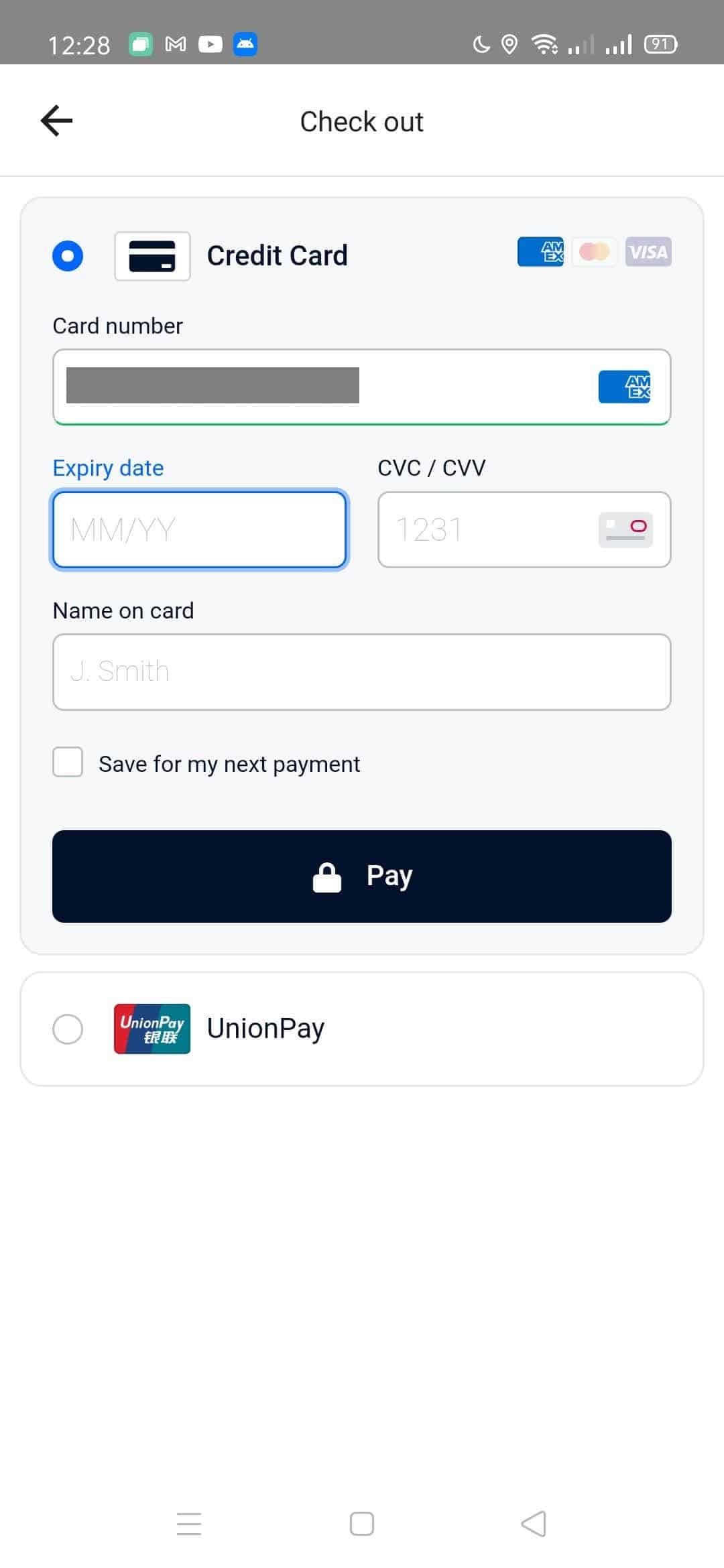The image is a screenshot from a mobile device displaying a checkout page. At the top, there is a gray bar extending across the full width of the screen, featuring icons on the upper left and upper right corners. The title, "Checkout," is prominently displayed in black font within the white background below the gray bar. To the left of the title is a black back arrow button. Adjacent to that, after a small space, is a vertical gray separator line followed by another space. Below this section, there is a gray box for inputting payment details, which include fields for entering a credit card number, expiration date, CVC/CVV code, and the cardholder's name. A checkbox option is available for saving this information for the next payment. At the bottom of the payment section, there is a prominent black "Pay" button. Below this section, there is another checkbox asking the user to "Check off Union Pay." The overall layout is clean and user-friendly, guiding the user through the payment process step-by-step.